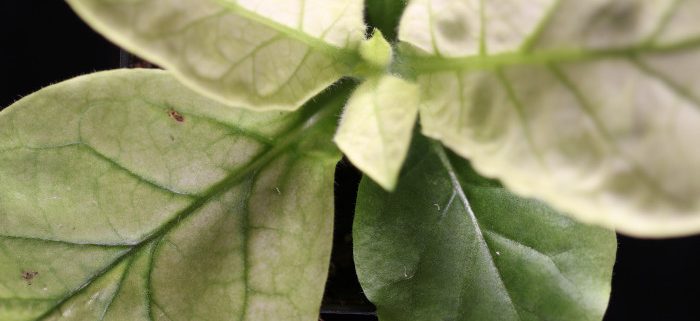This close-up photograph captures the intricate details of multiple green leaves set against a solid black background. The central focus is on four leaves, three of which exhibit a light green hue with dark green veins prominently running through them—one on the left side and two on the upper sections. The fourth leaf, located on the lower left, is a darker green. Small brown dots are scattered across the leaves, potentially indicative of mite activity. The background ensures no distractions, drawing attention solely to the leaves and their detailed textures, including one leaf that appears to have been bitten by an insect. The image primarily showcases the interplay of light and dark greens, accentuated by the stark contrast of the black background, to highlight the natural beauty and potential ecological interactions of the leaves.